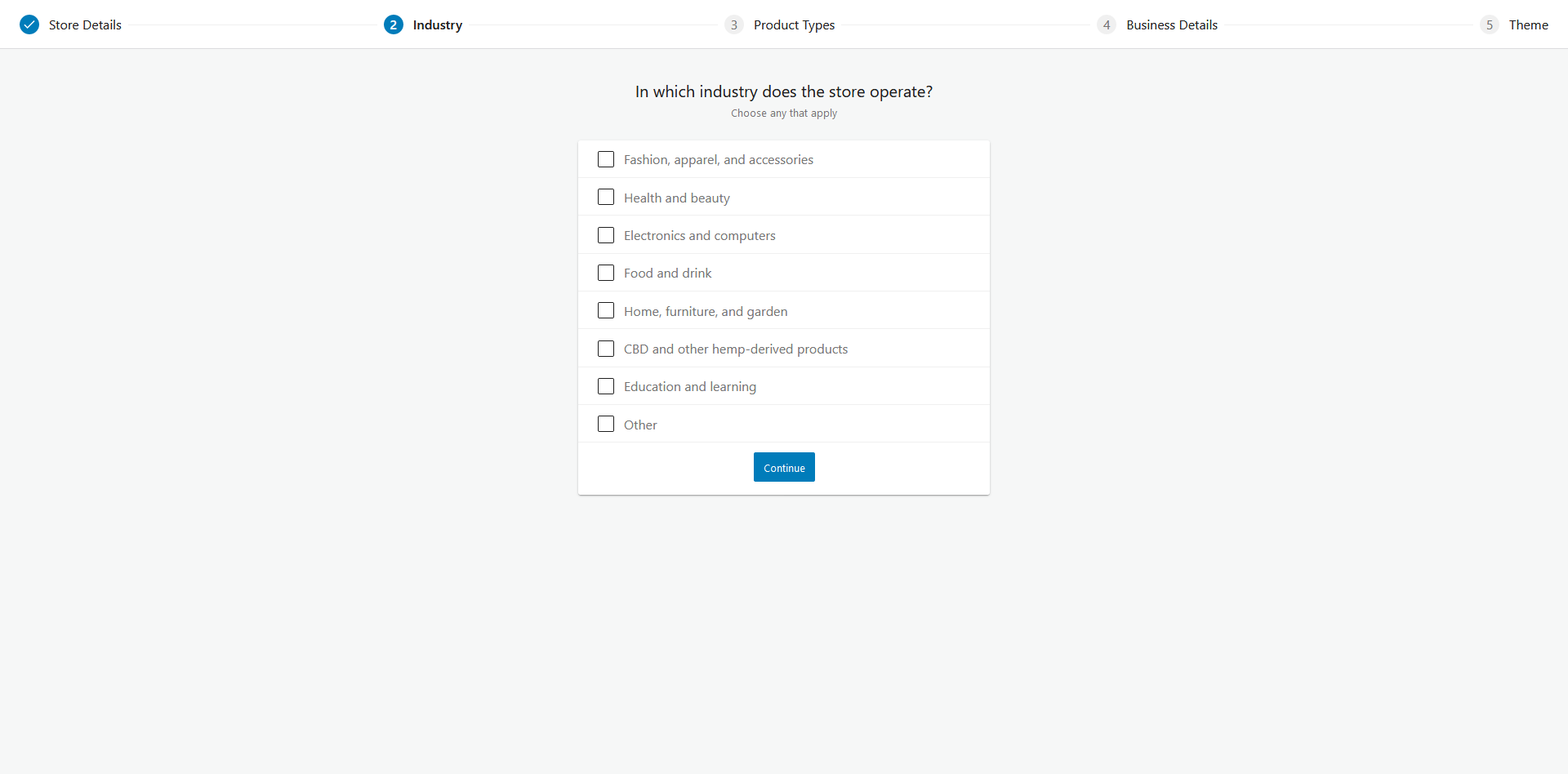Image Description: A screen capture from a desktop computer displays a user interface with a pale off-white background. At the top of the screen, five numbered menus are aligned horizontally from left to right. The first menu, marked by a blue circle with a white check mark icon, is labeled "Store Details" in black text. The following menus are titled "Industry," "Product Type," "Business Deals," and "Team," respectively.

Below these menus, there is a small form featuring multiple checkboxes which are currently empty. The form prompts the user with the question, "In which industry does the store operate? Choose any that apply." 

Four options are listed beside the checkboxes:
1. "Fashion, Apparel, and Accessories"
2. "Health and Beauty"
3. "Electronics and Computers"
4. "Food and Drink"

The interface appears to be part of an application or platform used for managing store-related information, likely aimed at categorizing stores based on the industries they operate in.